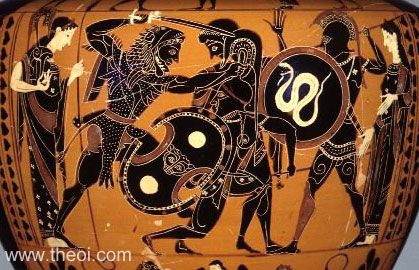This close-up photo showcases the side of an ancient Greek vase, presented by www.theoi.com, prominently featuring a detailed depiction of ancient warriors engaged in battle. The scene is rendered in black and white with some dark brown accents against the vase's striking orange background. Four warriors, illustrated with a high degree of intricacy, dominate the scene with their swords, spears, shields, and helmets. Notably, one of the figures wears an animal pelt on his head, suggesting a more barbaric persona. Each warrior is deeply engaged in the tussle, highlighting the intense nature of the conflict. On either side of the combatants, two women stand as onlookers, adding a unique dimension to the tableau. The artists have paid particular attention to certain light-colored elements, such as the faces, arms, and hands of the figures, as well as a distinct snake motif on one of the soldiers' armor. This ancient piece of art not only captures a moment of fierce battle but also reflects the artistic techniques and cultural storytelling of the time.